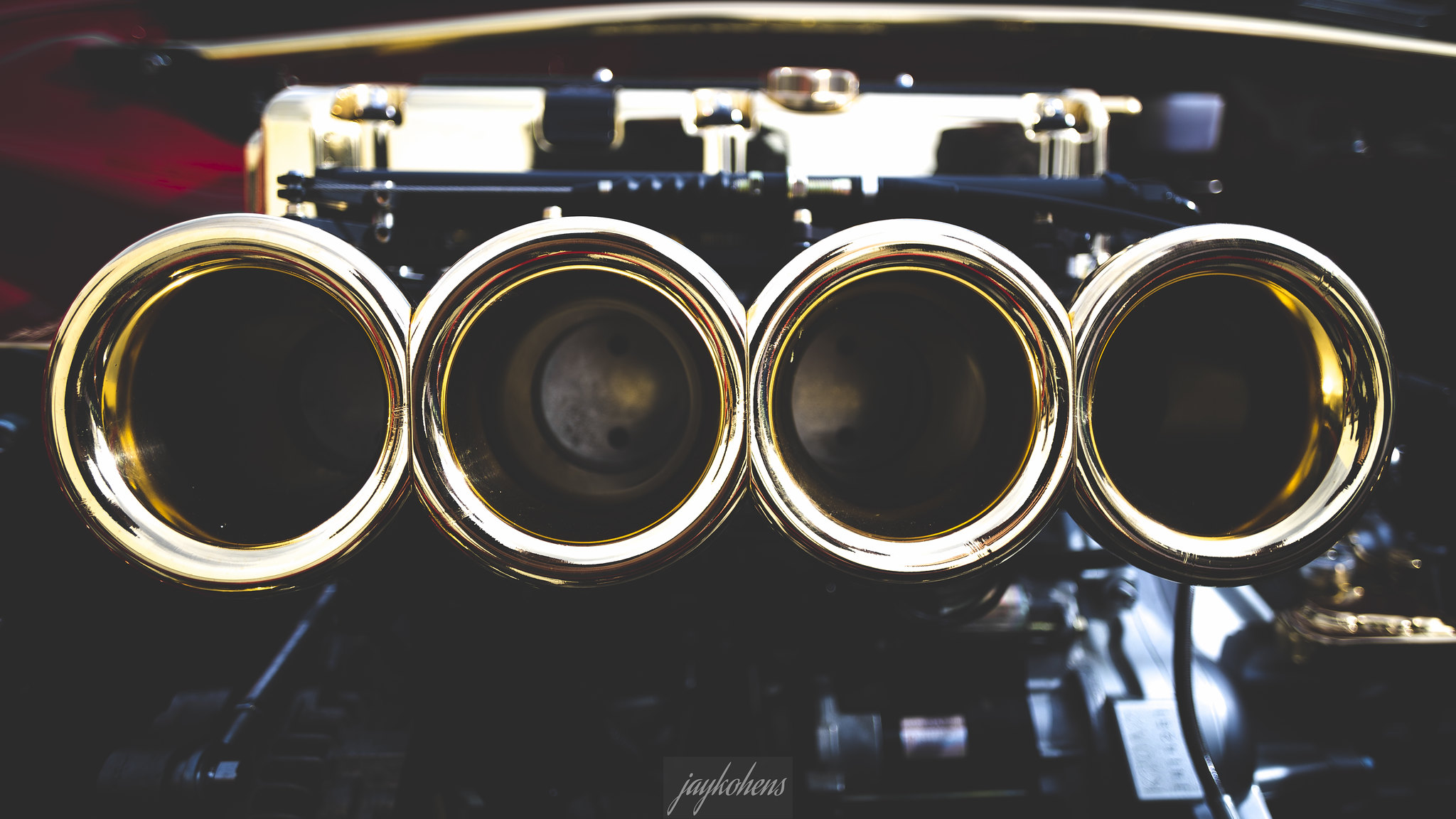This extremely close-up, color photograph in portrait orientation showcases a detailed, yet ambiguous mechanical or possibly musical object. Dominating the image are four golden, cylindrical ends, prominently displaying their circumferences. The middle left and right cylinders reveal their interior metal plates, featuring drilled holes and shadowy depths. These elements evoke the appearance of front air intakes akin to those on a supercharger of a sports car, such as a Mustang.

The backdrop, though out of focus, consists of a mix of red, blue, and white colors, contributing to the image's obscurity. Accentuating the scene are additional golden highlights, a black rod, and mechanical components, hinting at a complex assembly. At the bottom center, a small black plate with metallic white cursive text reads "Jay Coen's," possibly identifying the artist or the subject's brand, though its exact significance remains unclear. The photograph's tight framing and focused detailing on the brass-like cylinders, set against the blurred background, create a mysterious and visually intriguing composition.